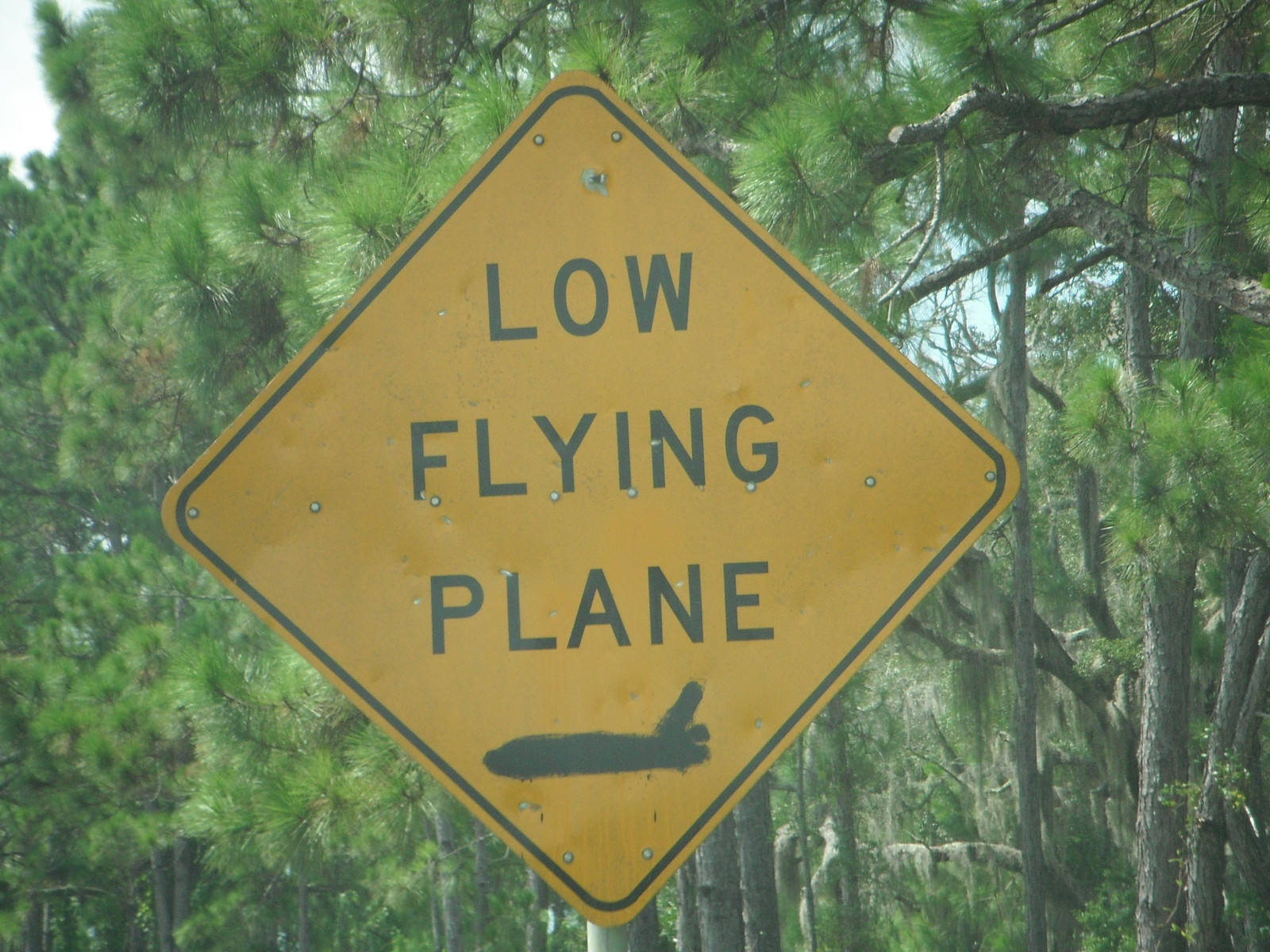In the foreground of this image stands a distinctively yellow street sign, prominently featuring a bold, black border that enhances its visibility. The sign, oriented diagonally in the frame, bears a clear warning message: "Low-Flying Planes." Beneath this text, a black silhouette of an airplane further illustrates the caution advised. The lettering on the sign is rendered in block-style fonts, making it easily readable. The backdrop of the image is a lush expanse of greenery, dominated by what appears to be dense foliage of pine or evergreen trees, reminiscent of the verdant landscapes commonly found in the Southern United States. This natural setting contrasts sharply with the bright yellow of the warning sign, drawing immediate attention to its urgent message.